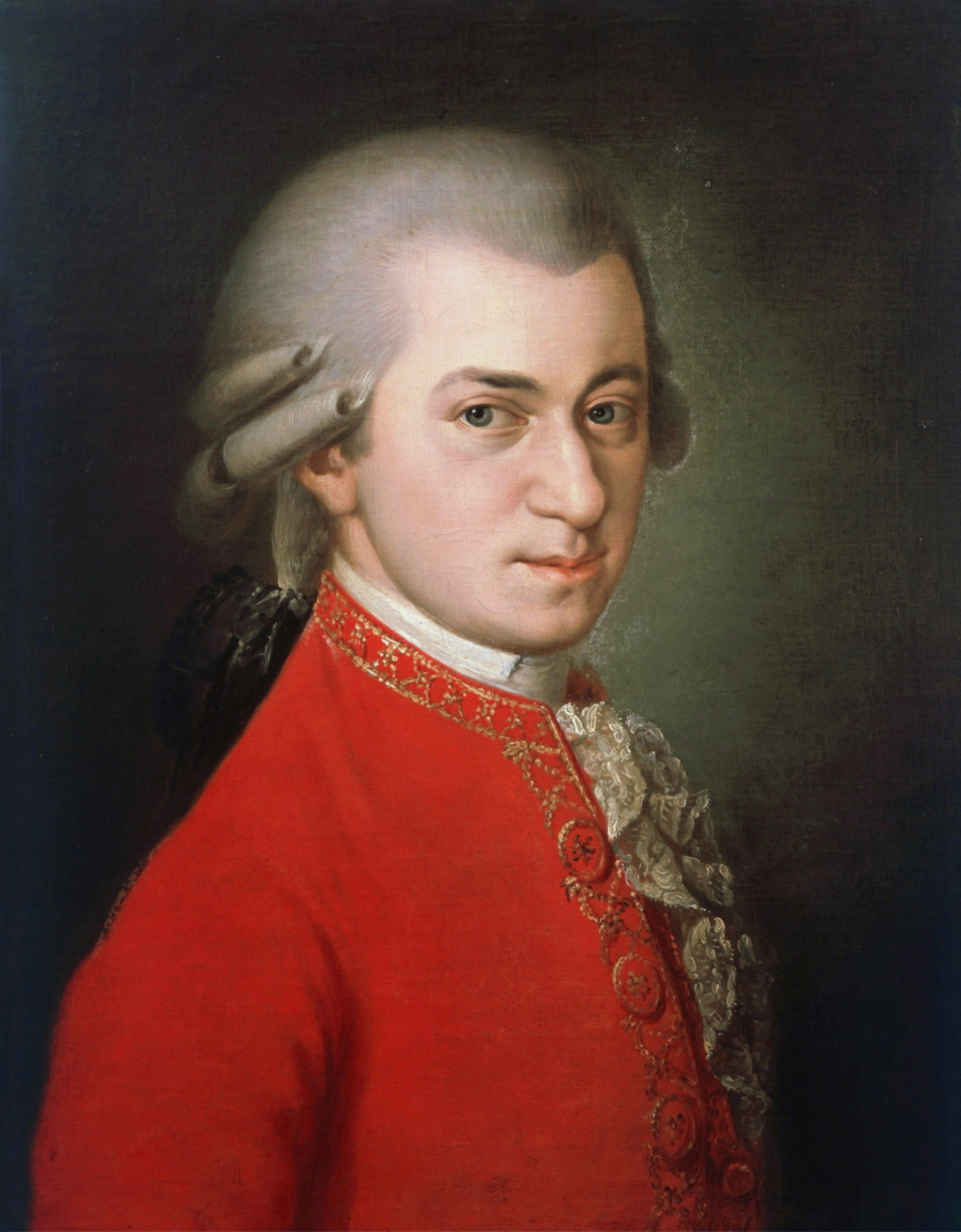The image is a detailed oil painting of the musical composer, Mozart. This close-up illustration captures him facing right with his head turned towards us, showcasing his refined, young Caucasian features with striking blue eyes, darker brown eyebrows, a well-defined nose, thin pinkish lips, and rosy cheeks. He dons a classic white wig with cylindrical curls at the sides and short black ribbons adorning a ponytail at the back. Mozart is dressed in a richly decorated red coat with intricate gold embroidery and large decorative buttons. A white ruffled handkerchief with detailed frills adorns his chest, beneath which peeks out a white collar. The painting employs a dark background with a subtle green glow emanating from the figure, creating an illuminating effect around him and gradually fading into black towards the corners, adding a dramatic contrast to the portrait.